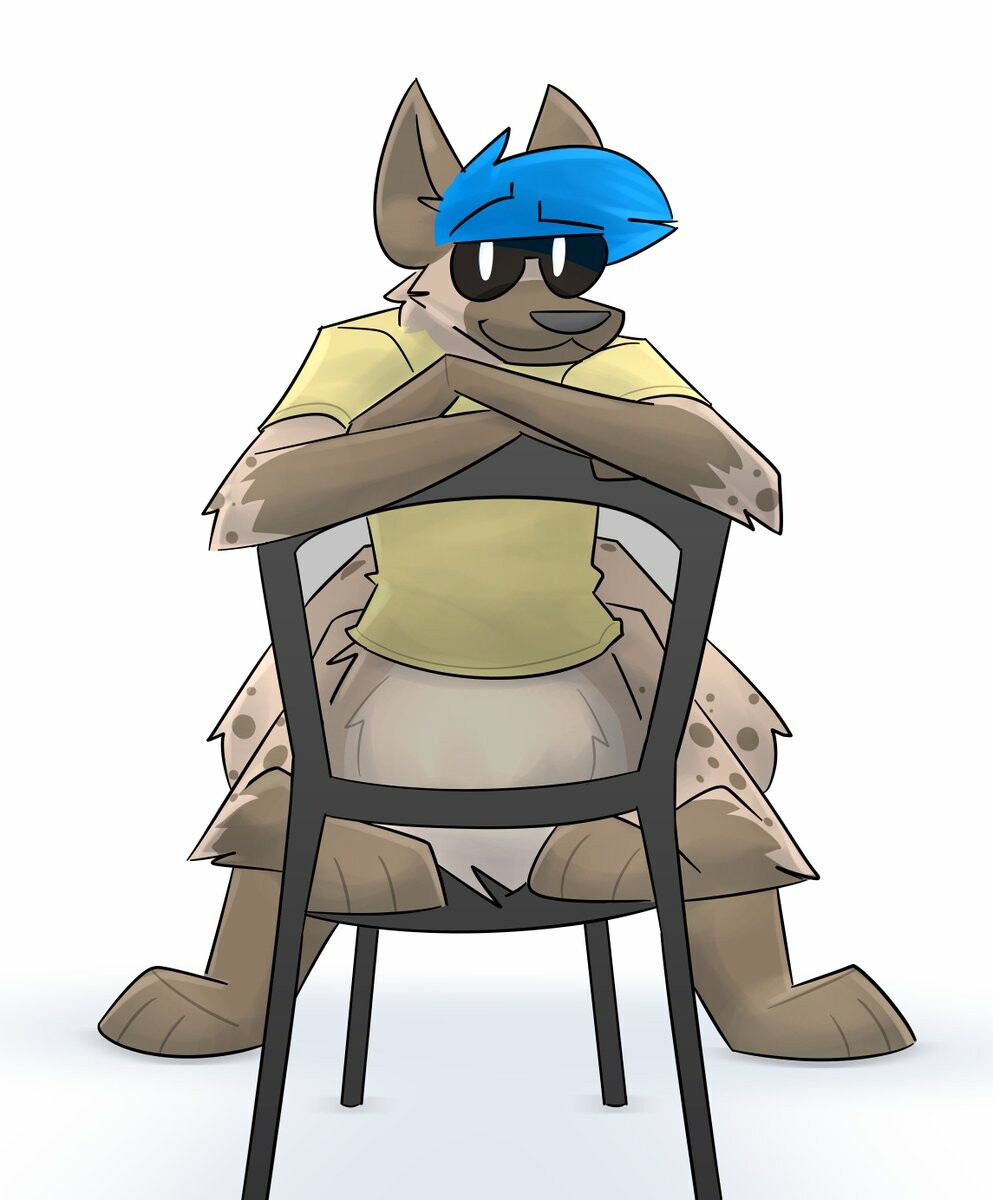In this artistic cartoon sketch against a light gray or almost white background, a character that resembles a brown and tan kangaroo or dog with human features is depicted sitting backwards on a gray or wooden chair with four legs and an open back. The character's arms are folded across the top of the chair, and its legs are spread on either side. It dons a yellow shirt, black sunglasses, and a blue visor, with two large brown ears peeking through the visor. The character has a dark brown or black nose and appears to have a subtle smile on its face. The feet and parts of the body are notably brown, complementing the animated and whimsical style of the drawing.